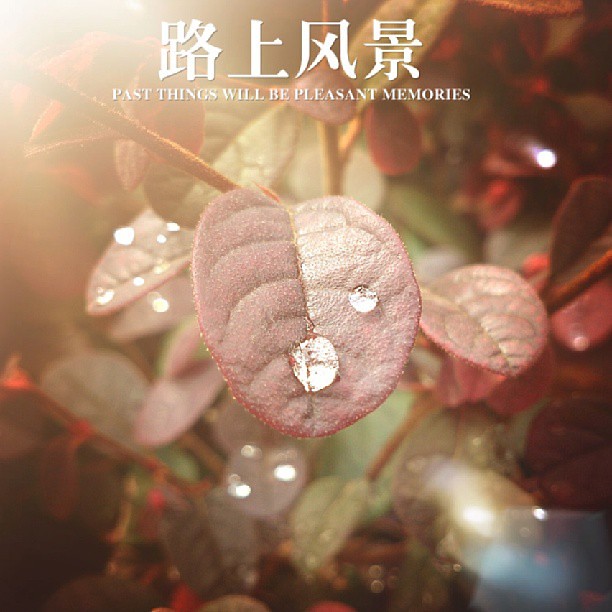The image is an inspirational photograph featuring a close-up of a prominently placed pinkish-reddish leaf with a velvety texture and two water droplets, one larger and centrally located, and a smaller, lighter one. Surrounding this central leaf are more medium-sized leaves on reddish-brown branches, creating a rich and layered composition. Some of these surrounding leaves also bear sparkling water droplets, which are translucent and reflect light, adding a visually appealing shimmer. The background is blurred, providing depth and highlighting the focus on the central leaf. At the top of the image, there are four large characters in what appears to be an Asian language, possibly Chinese, with a translation below in smaller white text that reads, "Past things will be pleasant memories." In the upper right corner, red leaves with a purple gleam are visible, with one specific water droplet reflecting light vividly. The bottom left corner contains a gray shadowy figure, adding a subtle, mysterious element to the composition.